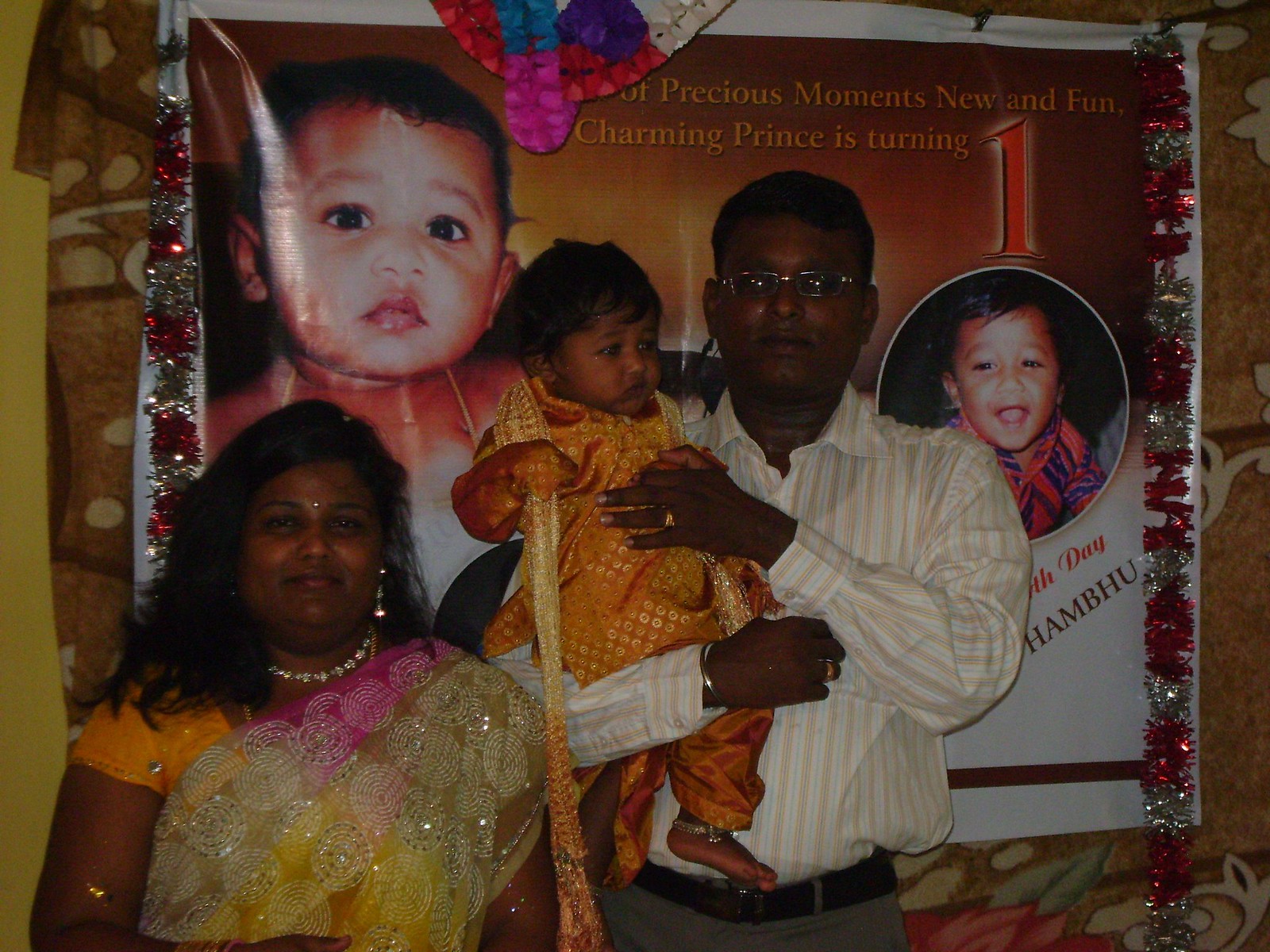The photograph captures a celebratory moment of an Indian family standing in a dimly lit room in front of a festive banner. The banner, attached to a yellow wall and decorated with red and gold tinsel, prominently features images of children and reads, "Precious moments, new and fun, charming prince is turning one," though parts of the text are cut off. 

The man, dressed in a white and yellow striped button-up shirt with gray pants, holds a small girl, about eight or nine months old, who is adorned in a colorful golden satin dress. The baby's dark hair and eyes match her dark skin, complementing the family's appearance.

To the man's left stands a woman in a traditional Indian outfit consisting of an orange top paired with a pink and yellow sari wrapped around her, her long black hair falling over a yellow wrap or sarong. She wears a pearl necklace and earrings, smiling moderately. The ensemble conveys a warm and vibrant celebration, likely a first birthday party for the young child.